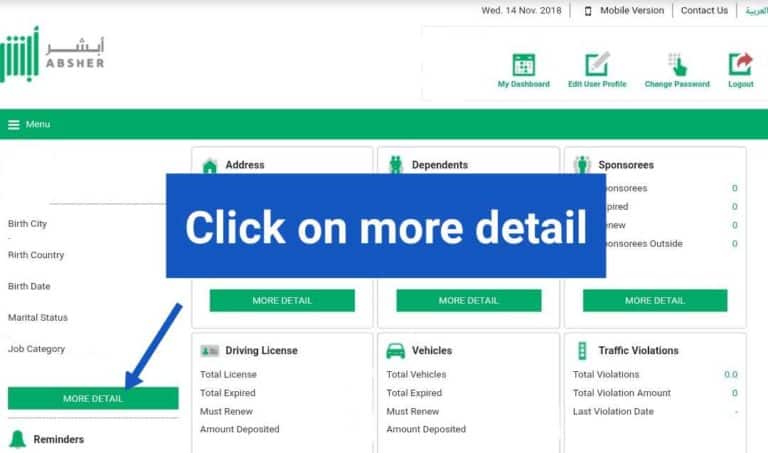The screenshot depicts a user interface from an institutional driver's license management system designed by Apture. At the upper left corner, the Apture logo is displayed in gray, accompanied by a green vertical line and dot motif. The top right corner features four main department selections: "My Dashboard," "Edit User Profile," "Change Password," and "Logout," each adorned with green and white icons, with the "Logout" option also marked by a red out arrow. Situated above these options, a section titled "Basic Site Information" provides the current date, confirms it's a mobile version, and includes "Contact Us" and a green icon.

Dominating the center of the page is a prominent blue pop-up button with the text "Click for more detail" in white, with a downward-pointing blue arrow guiding users towards a submenu on the right side of the page. This submenu, located on the far right column, comprises primary user details such as birthplace (city and country), birth date, marital status, and job category. Further down this column, a small green bell icon followed by dark text labeled "Reminders" can be found.

The main body of the page is organized into six distinct sections: "Address," "Dependents," "Sponsorees," "Driving License," "Vehicles," and "Traffic Violations." These sections are arranged in three vertical columns and each features a green button offering the capability to access more detailed information.